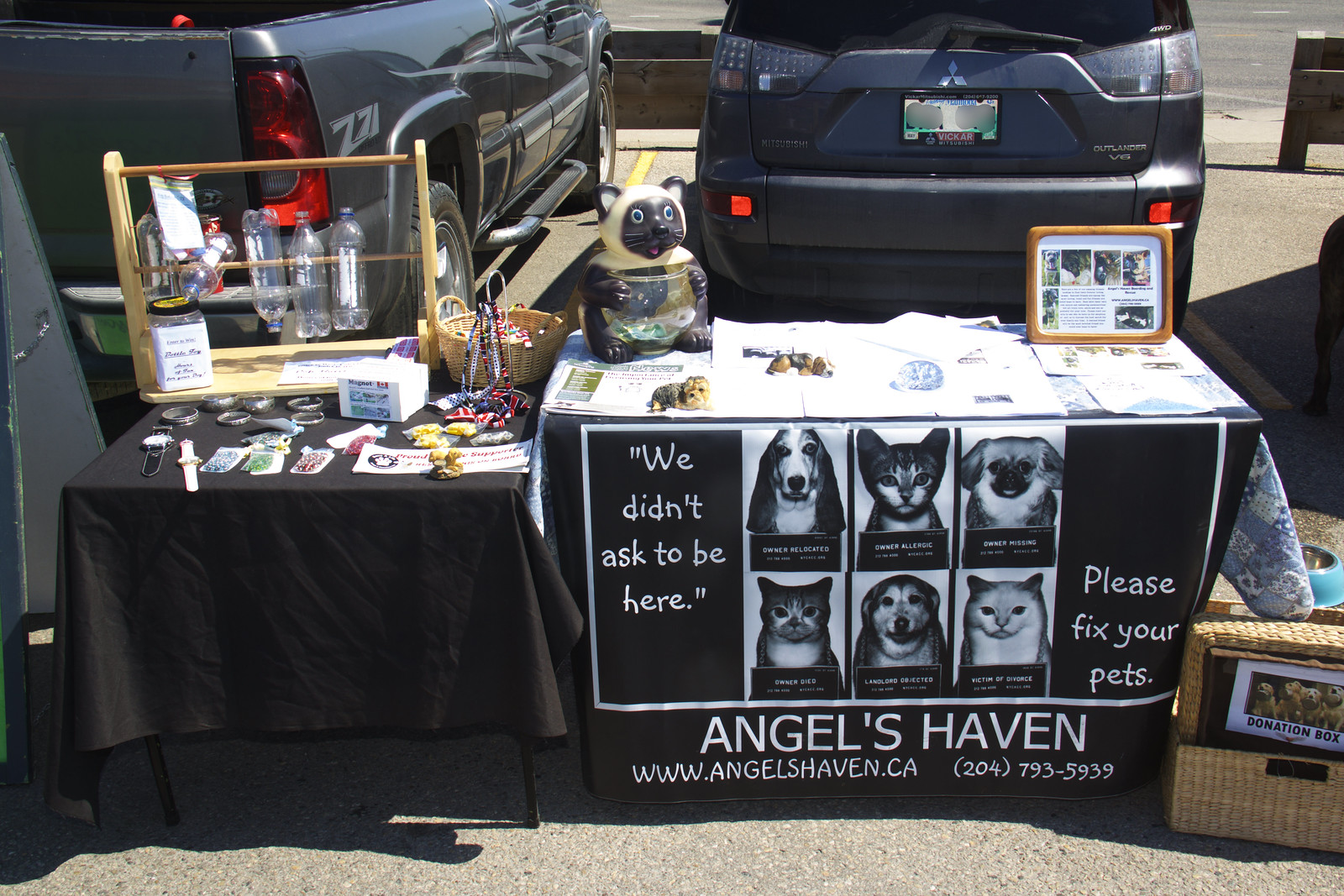The image captures an outdoor booth set up, likely at a craft fair or similar event, designed to educate people about fixing their pets. The main focus is the table draped in a black cloth, positioned centrally. On the table, a variety of objects are displayed: jewelry, papers, water bottles, and decorative figurines of cats and dogs. A poignant sign features images of cats and dogs with the text, "We didn't ask to be here. Please fix your pets," accompanied by the logo and website for Angel's Haven (www.angelshaven.ca). Nearby, a wicker basket marked as a donation box and filled with trinkets and perhaps jewelry, underscores the booth's mission. Behind the table, the backdrop includes parked cars, with visible details such as the gray vehicles, a yellow parking line, and possibly the rear of a van or truck. The colors throughout the scene include varying shades of gray, blue, black, tan, white, green, and red, adding vibrancy to the setup. This booth, with its neatly arranged pamphlets and framed photographs, emphasizes the urgency and importance of pet care and responsible ownership.